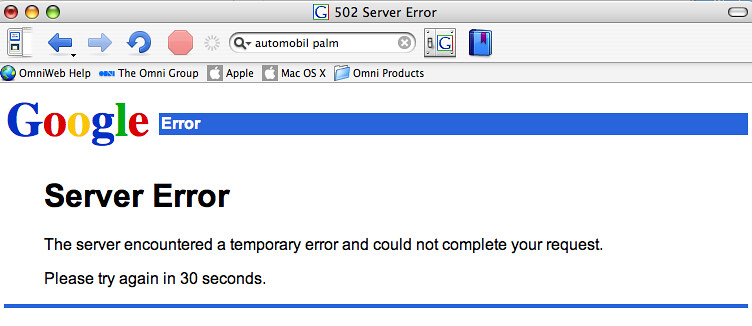The web page displayed is a Google search window featuring an old Google logo with the iconic letters: "G" in blue, "O" in red, another "O" in yellow, "G" in blue, "L" in green, and "E" in red. Centrally positioned near the top, the page announces a "502 Server Error" indicating that the server encountered a temporary problem and could not complete the requested action. The message advises to "please try again in 30 seconds." In the top left corner are three circular icons colored red, orange, and green, arranged from left to right. The background is white with black text. Additional elements include a horizontal thin blue line at the bottom and various interface bars for the Omni Group, Apple, MacOS, and Omni Products near the top.